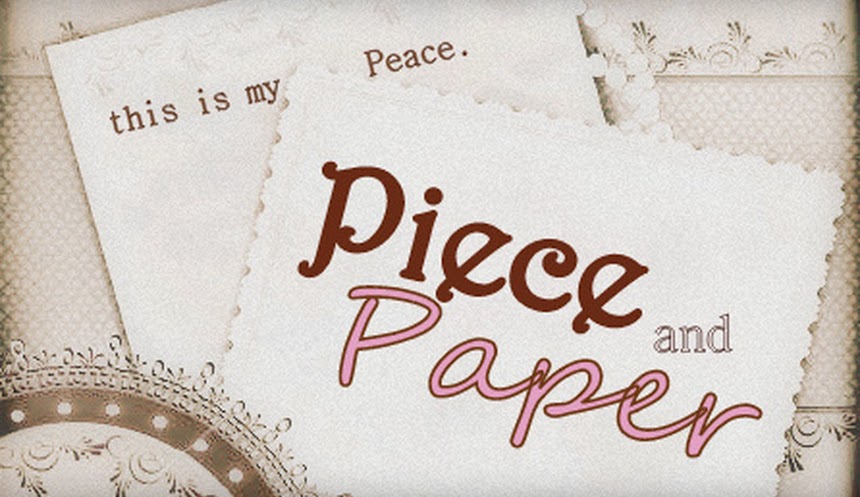In the image, there's a promotional advertisement featuring intricately designed stationery. The central piece of paper prominently displays "piece" in a dark brown, "and" in a light color, and "paper" in pink cursive with a brownish outline. The paper sits atop another that reads "this is my piece" in straightforward text. Both pieces are placed on a decorative background with an ornate, swirling border in shades of beige, gray, and off-white, resembling cracked eggshells. The left side features a half-circle doily design with similar swirling patterns. The overall color palette includes rusty browns, pinks, beiges, and whites, suggesting an elegant, possibly handmade or artisanal theme, likely related to a high-quality stationery or party favor business.